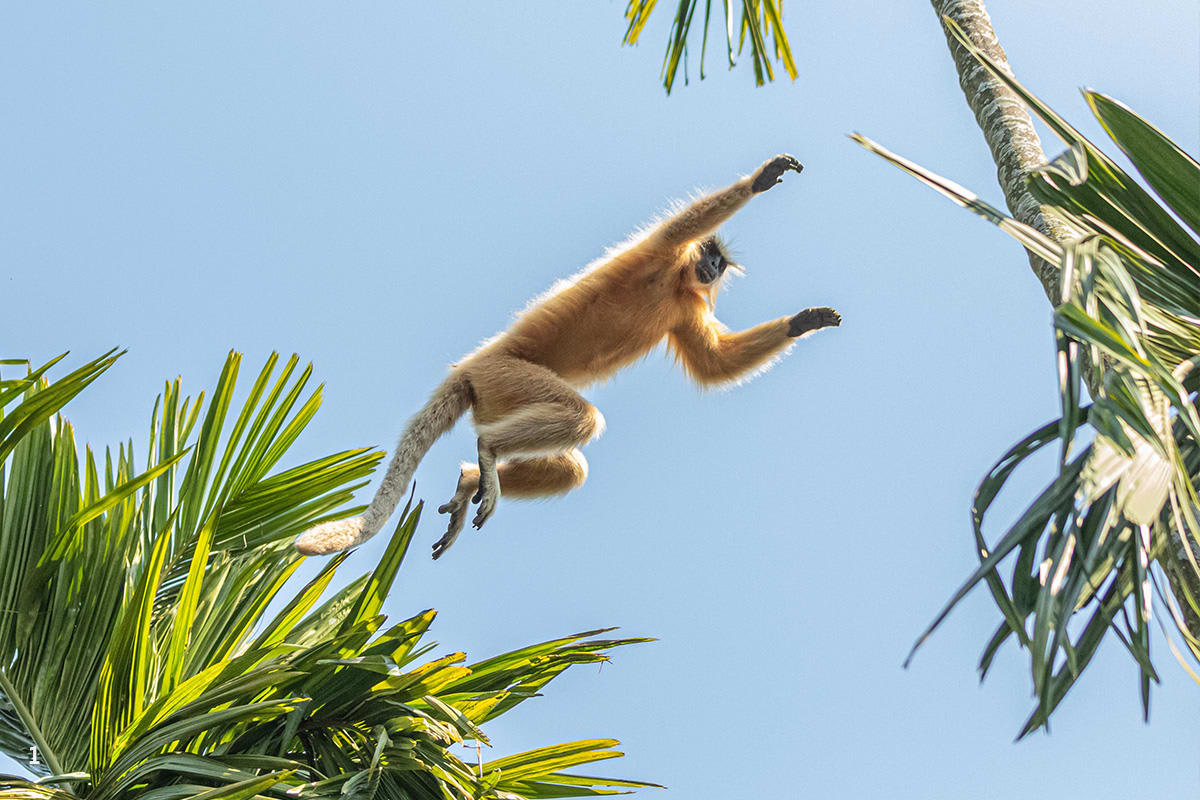The photograph, which resembles an in-game screenshot due to its vivid coloration and detailed scenery, captures an action shot of a monkey in mid-flight against a clear, powder blue sky. The scene is set in daylight, emphasizing the bright, sunny atmosphere. On the left, only the very top of a palm tree with green and yellow leaves is visible. To the right, we see just the middle section of a tall tree characterized by white and brown bands and large leaves.

The monkey, with its striking ginger-colored fur, stands out against the backdrop. It has a black face, black palms, and the soles of its feet are black as well. Its long tail, furry but not fluffy, trails behind as it leaps. The monkey's body is dynamically posed, with arms fully outstretched in a Superman-like manner and legs bent, showing the energy of its push-off. This captivating snapshot perfectly freezes the moment of the monkey's daring jump from the left treetop to the taller tree on the right.